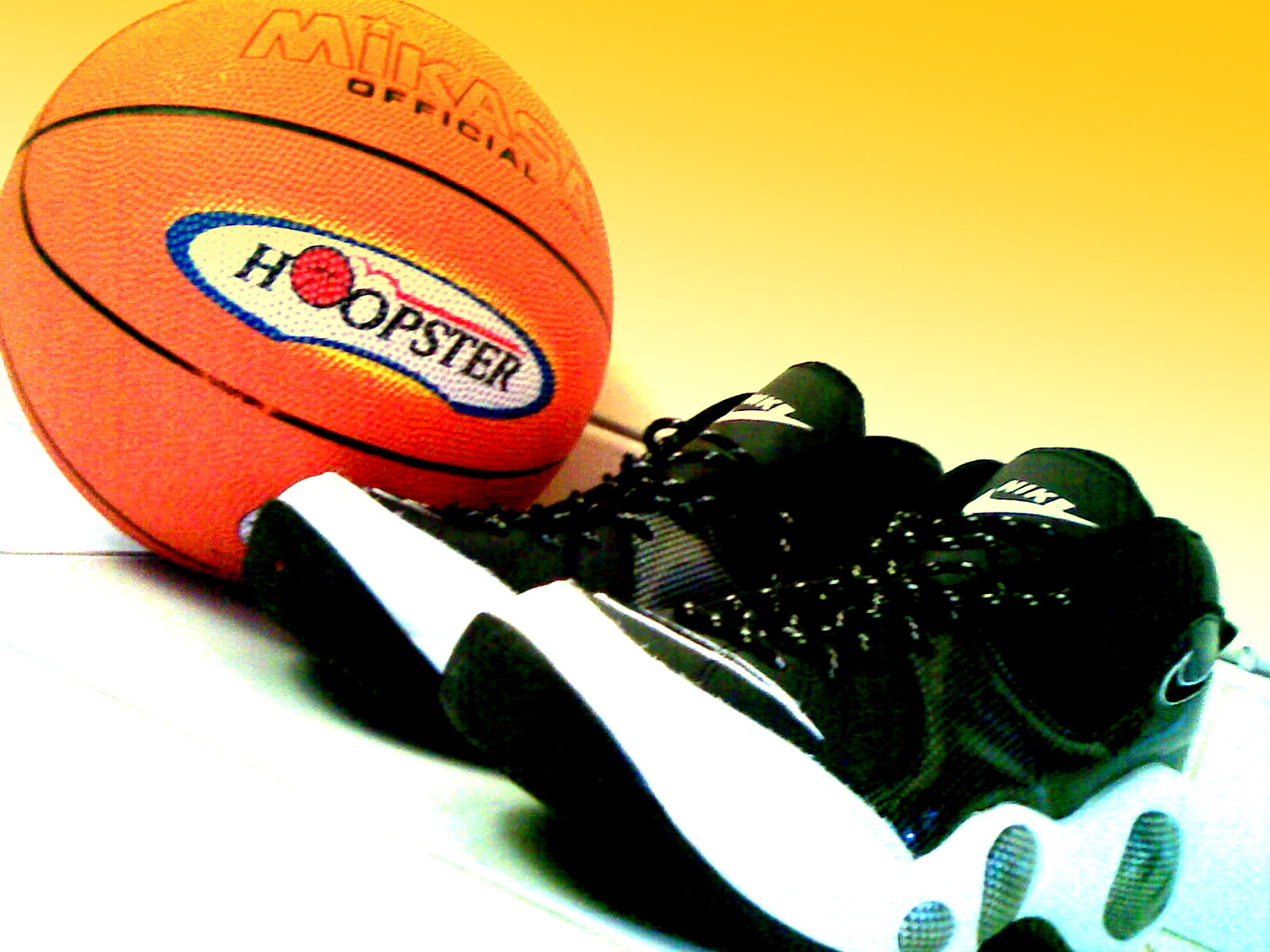In this photograph, we see an orange Mikasa basketball and a pair of black and white Nike basketball sneakers. The background features a yellow wall and a white surface. The basketball, positioned in the top left corner, prominently displays the brand name "Mikasa" in orange letters with "Official" written below in black. The ball also features a circular logo with yellow and blue outlines, and a white background containing the word "Hoopster" in black letters, where the first "O" has a red center. Adjacent to the basketball, in the bottom right, are the Nike sneakers. These sneakers are black with white accents, including a white Nike logo and swoosh on the tongue and a black swoosh on the side. The photograph emphasizes the detailing on both the basketball and the sneakers, showcasing their distinct brand elements and colors.